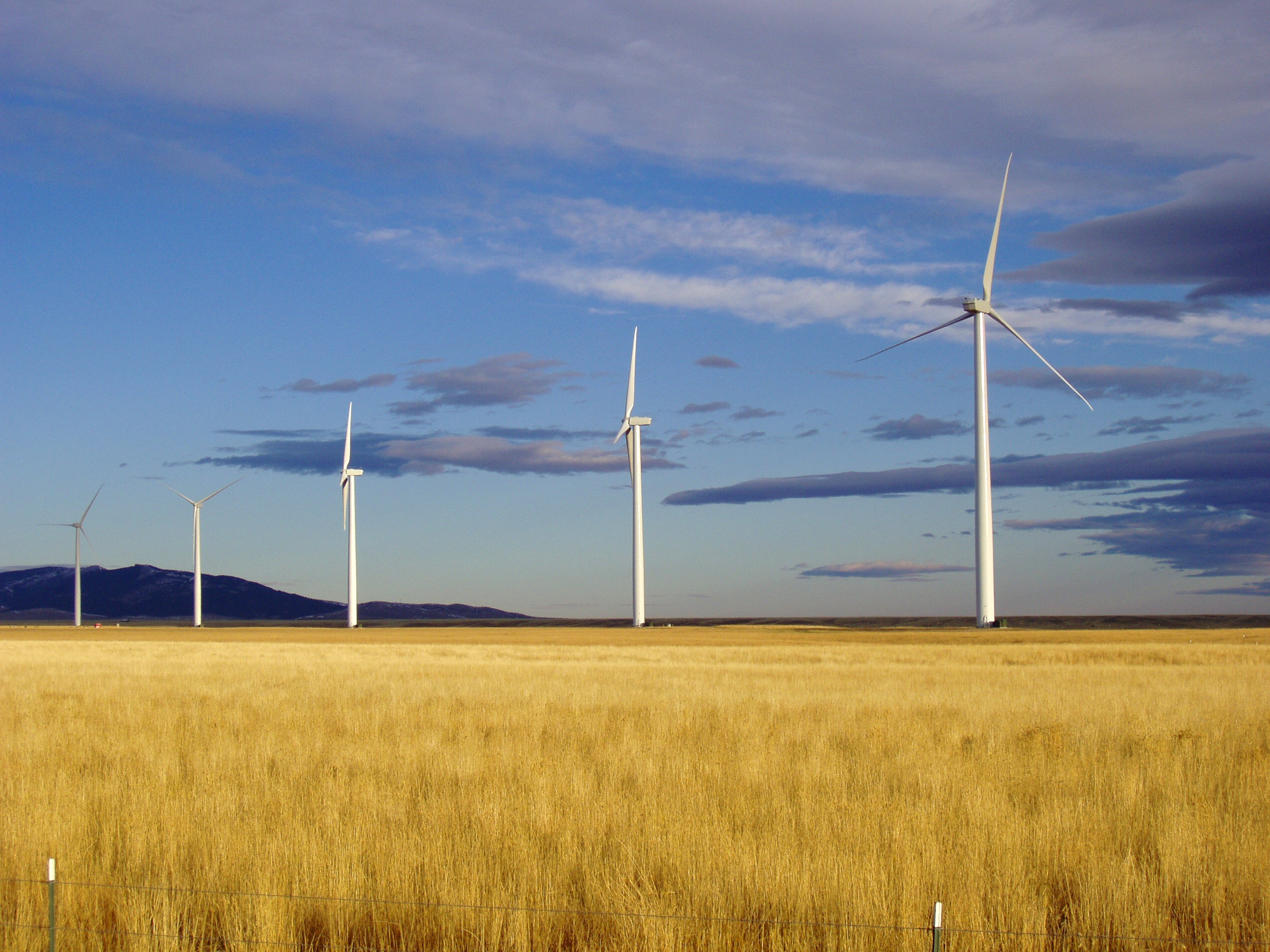The image captures a vast, golden field that resembles the color of wheat, evoking a desert-like landscape found in regions like California or Arizona. Prominent in the photo are five towering white wind turbines, each with three distinct, triangular blades designed to catch the wind. The sky overhead is a striking blue, punctuated by patchy clouds, creating a picturesque setting. In the foreground, a modest chain-link fence encloses the area, adding a layer of depth to the scene. This expansive, sunlit field dotted with wind turbines is reminiscent of the open spaces often seen in Texas, painting a serene yet industrially active landscape.